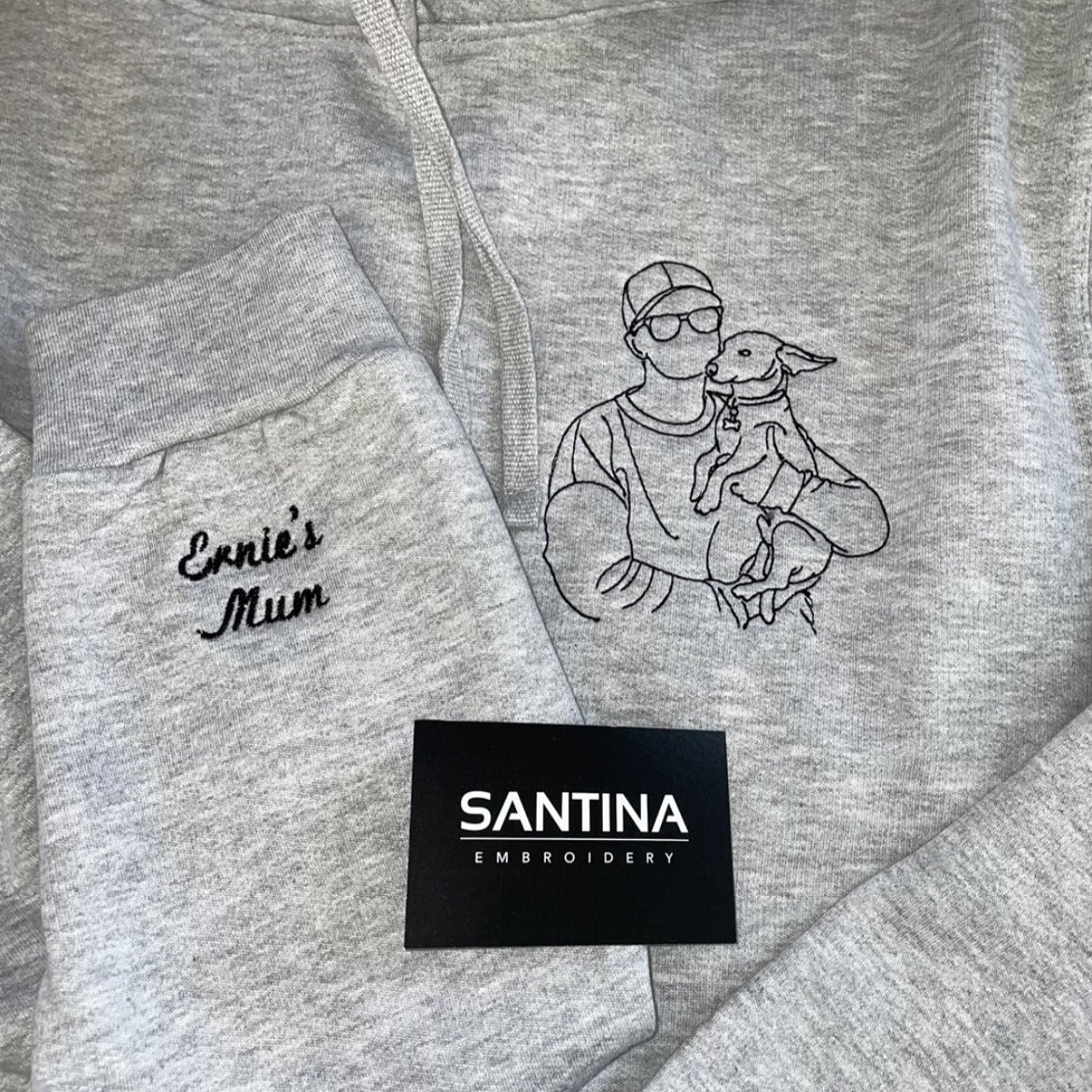The image depicts a heather gray hoodie made of soft material, with drawstrings hanging from the neck. The hoodie prominently features detailed embroidery work. On the chest, located on the upper right side, there is an outlined logo of a man wearing a baseball cap and glasses, holding a small dog in his left arm. The dog, which seems to be a Jack Russell, has a collar with a bone. Additionally, one sleeve displays the inscription "Ernie's Mum" in a European script style. A black card sits atop the hoodie, displaying the words "Santina Embroidery" in white letters, emphasizing the hoodie as an advertisement piece for the embroidery company's craftsmanship, showcasing both the text and logo embroideries.